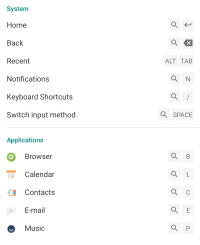The image is a low-quality, blurry screenshot of a mobile phone's settings menu, characterized by its indistinct white background. Despite the poor resolution, the menu items are presented in a black font. The settings list includes: "System", "Home", "Back", "Recent", "Notifications", "Keyboard Shortcuts", and "Switch Input Method". To the right of each item, various icons are visible: 

- "Home" is accompanied by a magnifying glass and an arrow icon.
- "Back" has a magnifying glass and an X icon.
- "Recent" is marked with an Alt and Tab icon.
- "Notifications" display a magnifying glass and an N icon.
- "Keyboard Shortcuts" feature a magnifying glass and a slash icon.
- "Switch Input Method" shows a magnifying glass and a space icon.

Below these items, separated by a black line, is another section labeled "Applications". This section includes: "Browser", "Calendar", "Contacts", "Email", and "Music", each represented by distinct icons to the left:

- "Browser" is marked by a red circle.
- "Calendar" is indicated by a calendar page icon.
- "Contacts" is represented by a human silhouette icon.
- "Email" features a piece of paper icon.
- "Music" is symbolized by a record icon.

The overall image appears cluttered and visually unappealing due to the blurriness and low quality.